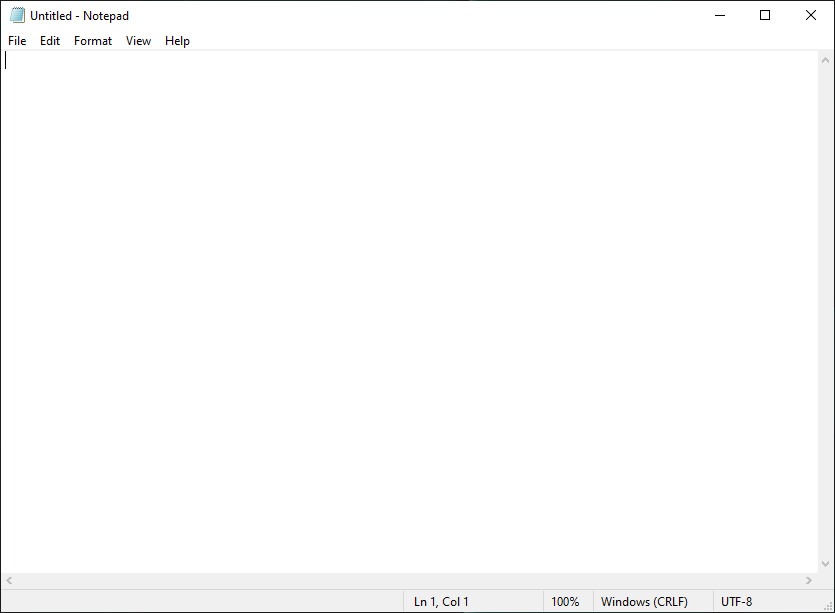The screenshot depicts a basic Notepad application interface. The main window is a large black-outlined square. In the top left corner, there is a small icon resembling a notepad, beside which is the title "Untitled - Notepad." 

In the upper right corner, there are three familiar window control buttons. The first is a horizontal line, which lets you minimize the window without closing it. Next to it is a hollow square icon that allows you to maximize or resize the window. Lastly, there is an X button to close the application entirely, taking you back to the desktop or another open application.

Directly below the title bar, there is a menu bar with five dropdown options: File, Edit, Format, View, and Help. These tabs let you navigate and perform different actions within the Notepad application.

The cursor is positioned at the very top of the text area, ready for typing beneath the File menu option on the left-hand side. The interface is clean, straightforward, and ready for the user to begin creating or editing a text document.